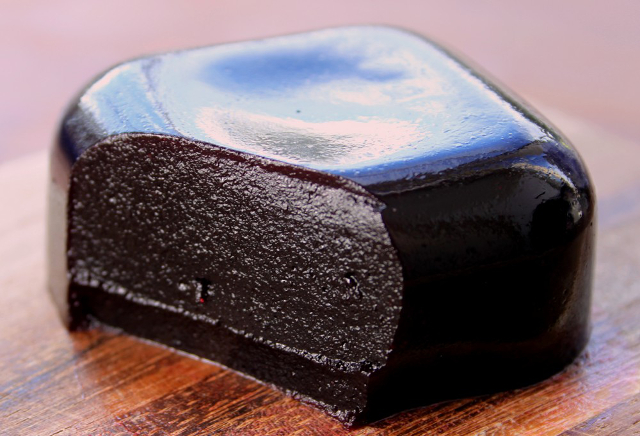This horizontal rectangular image depicts a black object with an unusual shape, placed on a mahogany wooden table. The table's wood grain is clearly visible in the foreground but fades to a lighter area in the background where the grain is less discernible. The object, likely made of black onyx stone, features a unique form resembling a square with a cut-off corner. It has a shiny, reflective surface with light bouncing off the top, giving it a slightly blue hue. The front face with the truncated corner is also shiny, while the exposed, textured interior on the left side contrasts with the smooth exterior, suggesting it might be a broken or cut piece. The overall composition and reflections on the object create a rich interplay of textures and light.